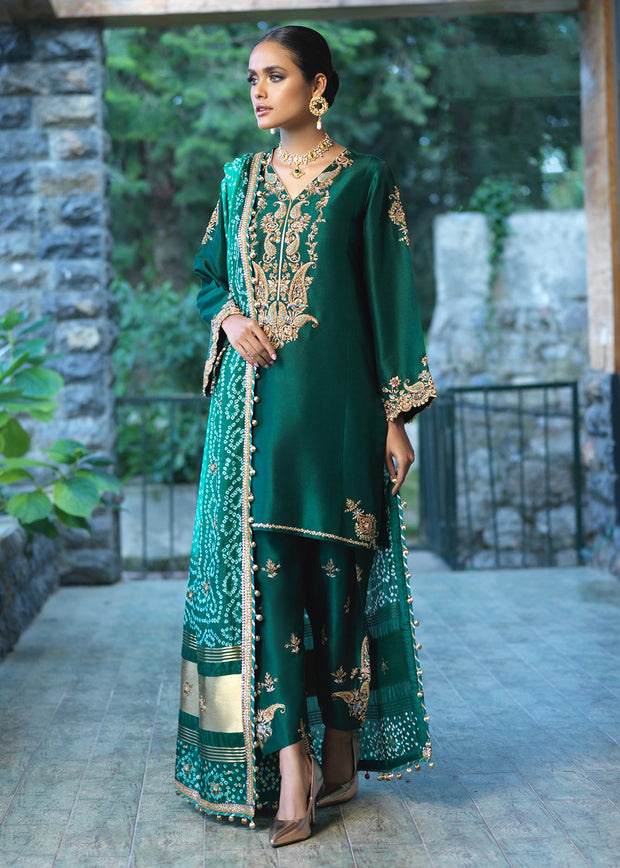In this captivating image, a young South Asian woman stands with an air of grace and poise on a stone terrace, surrounded by lush greenery and a waist-high black gate. She is dressed in a stunning traditional Indian outfit featuring a harmonious blend of dark kelly green, lighter green, and rich gold tones. Her attire includes an intricately decorated tunic with embellishments down the front and on the sleeves, which are designed to mimic lace. The tunic is complemented by tight green pants that end at her ankles and a long, elegantly draped wrap that reaches almost to the ground. She completes her look with gold high-heeled shoes.

Her hair is parted in the middle, slicked back, and styled into a tight bun, accentuating her refined features, which include a medium complexion and skillfully applied makeup. She accessorizes with large, gold medallion-like earrings adorned with dropped pearls and a thick gold necklace featuring a prominent green stone at its center, accompanied by smaller green stones throughout.

The woman gazes thoughtfully to her right, exuding a serene demeanor. The luxurious satin-like material of her outfit, embellished with gold accents, enhances the elegance and opulence of the ensemble, making it clear that this is a high-end and sophisticated look. The natural backdrop of trees and foliage further accentuates the timeless beauty of her traditional attire, creating a captivating and memorable portrait.